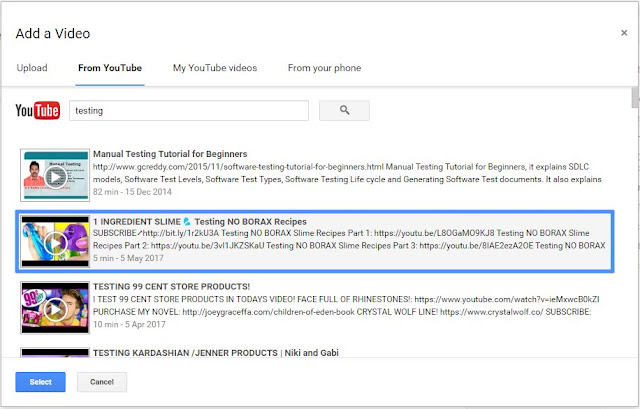This image depicts a YouTube webpage showcasing a selection of the user's uploaded videos. At the top of the page, visible text headers categorize the content. The lineup includes a variety of tutorials and product testing videos. Specifically highlighted are videos such as "Manual Testing Tutorial for Beginners," a "Slime Testing" video featuring no-borax recipes, and a series on "Testing 99 Cent Store Products." Additionally, there are more eclectic reviews like "Testing Kardashian Salt and General Products" and content from popular creators Nicky and Gabby. The layout and thumbnails serve to give viewers a visually engaging overview of the diverse video content available on this user's YouTube channel.